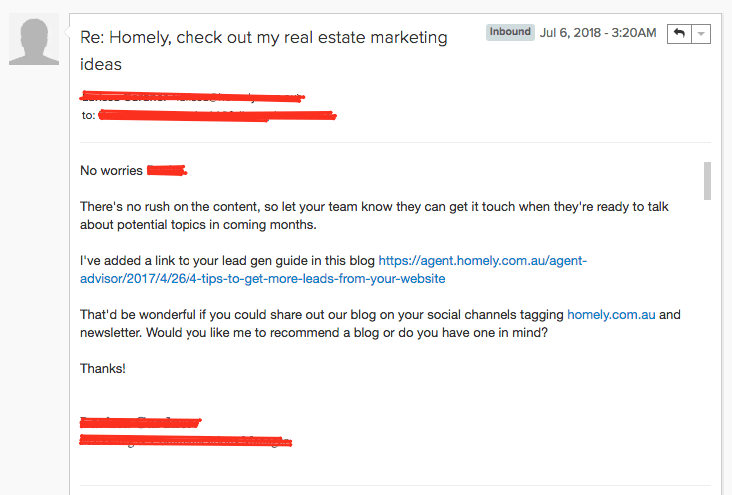Screenshot of an email received on July 6, 2018, at 3:20 a.m. The email is marked with an "inbound" tag. At the very top of the email, there's a grayed-out avatar resembling the silhouette of a person's head. Next to the avatar, within a cartoon-style thought bubble, is the subject line "RE: Homely Check Out My Real Estate Marketing Ideas." To the left of this bubble is a back arrow icon, indicating navigation options.

The sender's information and the email recipient's address are crossed out in red, making them illegible. Moving on to the body of the email, it begins with a casual "No worries [Name redacted]," followed by a detailed response about the lack of urgency on the content. The sender reassures the recipient that their team can reach out whenever they are ready to discuss potential topics in the upcoming months.

Included in the email is a hyperlink to a lead generation guide: [https://agent.homely.com.au/agent-advisor/2017/426/4-tips-to-get-more-leads-from-your-website](https://agent.homely.com.au/agent-advisor/2017/426/4-tips-to-get-more-leads-from-your-website), suggesting it be shared on social channels while tagging "homely.com.au." The sender also inquires if the recipient would like a blog recommendation or if they already have one in mind. Finally, the sender's name and title are also crossed out in red at the end of the email.